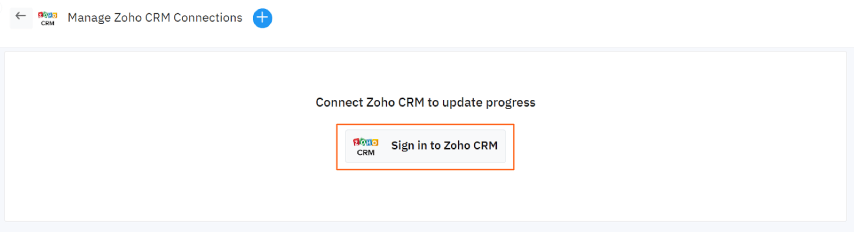**Detailed Caption:**

The image showcases the Zoho CRM connection interface designed with a minimalist and clean layout. In the top left corner, there's a small Zoho CRM icon next to the heading "Manage Zoho CRM Connections." Directly below, the main content area features a centered message that reads, "Connect Zoho CRM to update progress," along with a prominent button labeled "Sign in to Zoho CRM," which is outlined in orange. The background is predominantly white, contributing to the clean and straightforward design. Additional navigation elements include a back arrow, presumably for returning to the previous screen, and a blue plus icon, which might be for adding new accounts. This interface aims to facilitate user interaction, allowing them to seamlessly connect to their Zoho CRM account from the "Manage Zoho CRM Connections" tab.